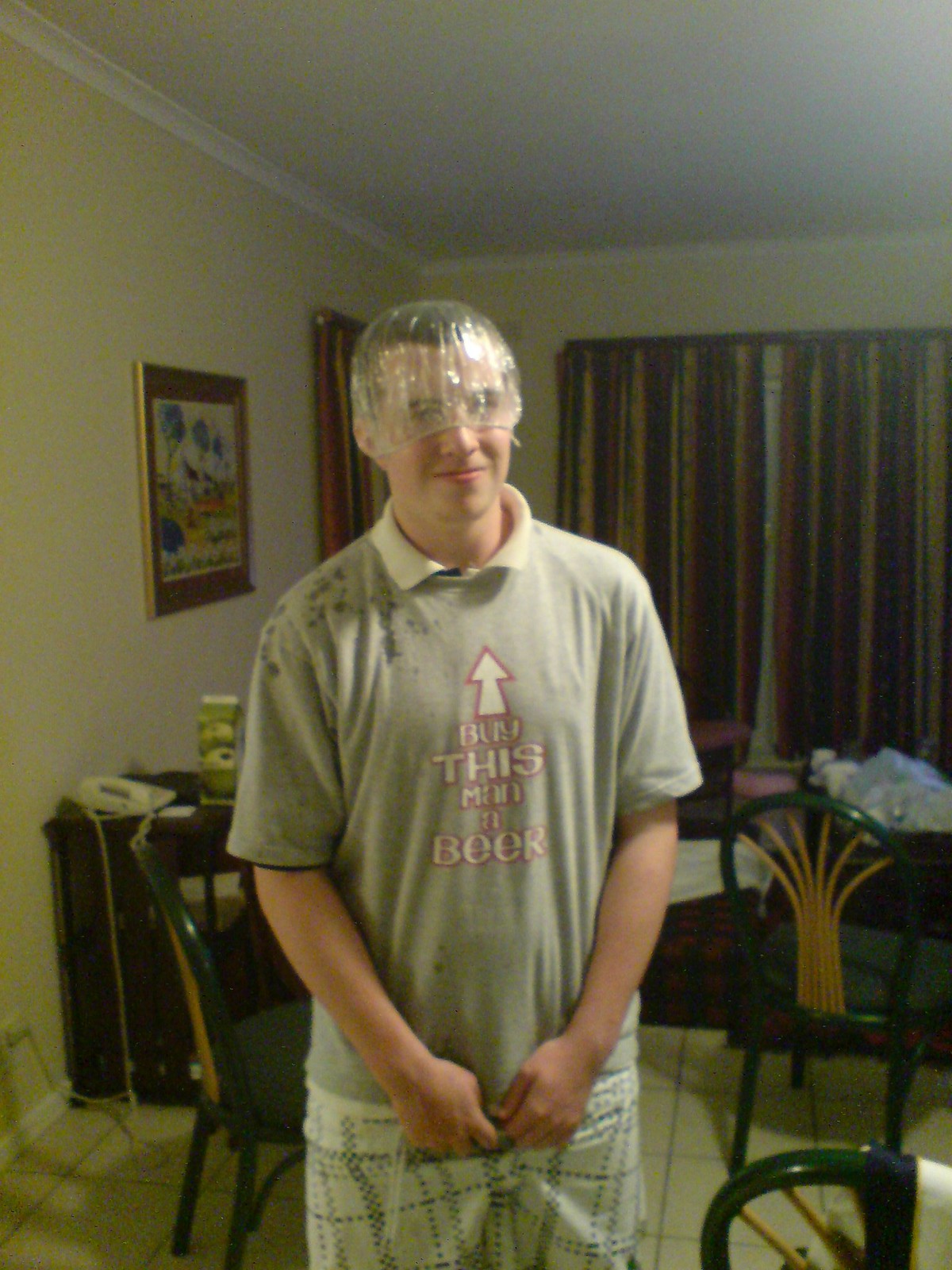In this detailed image taken inside a residential setting, potentially a living room or dining room, a man stands upright in the center of the room. He is dressed in a grey-colored t-shirt with a notable slogan that reads "buy this man a beer" in white letters with a pink outline, accompanied by an arrow pointing upwards towards his face. The man also wears dark-colored shorts and has his hands positioned over his crotch. Covering his head and eyes but leaving his nose and mouth exposed is a shower cap, giving him an embarrassed appearance. Over his right shoulder, there are marks resembling drops of water.

Surrounding the man, the room features three chairs that are primarily green with yellow parts and a window adorned with red, black, and yellow curtains. On the left side of the image, a picture frame hangs on the wall, and a small cabinet with a phone placed on top of it is also visible. The background includes kitchen tables and black chairs with natural wood spokes, contributing to the residential ambiance.